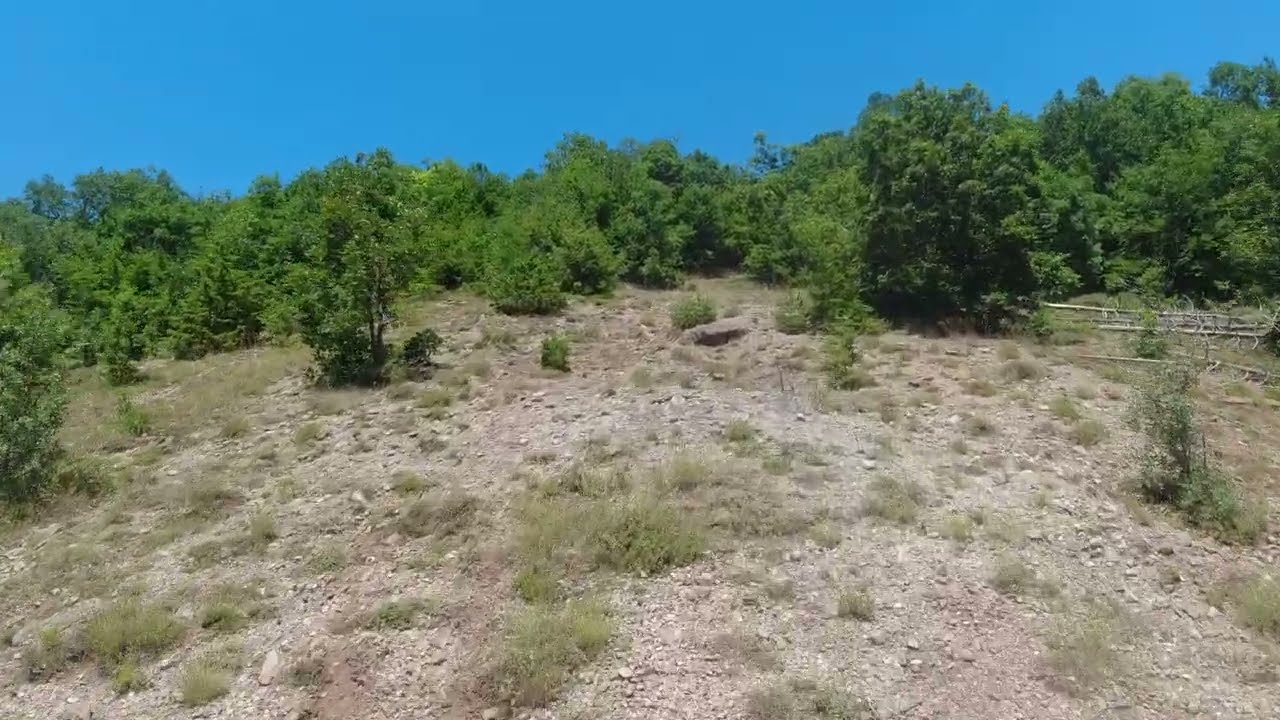The image showcases a vast outdoor landscape dominated by a dry, almost deserty expanse of light brown, dusty ground interspersed with beige and pale dirt patches. Scattered across the arid earth are numerous shrubs, some resembling tumbleweeds with their light yellowish-green hues, and brownish, sparse vegetation. Further into the middle of the image, lush and brilliant greenery takes over, with bright green trees and large shrubbery almost the size of trees creating a vivid contrast to the foreground. Towards the right middle, there appear to be thin tree trunks lying on the ground, seemingly rotting and devoid of branches or leaves. In the top right, partially obscured by large pine trees, sits the remnants of an old fence. The sky, occupying about the top third of the image, is a striking and uninterrupted electric blue, devoid of any clouds, enhancing the serene and untouched quality of the scene. The photograph, in landscape orientation, has a hint of drone photography, offering a broad, aerial view of the rugged rocky field with pine trees perched along a distant ridge. There are no people or animals present, providing a pure, unadulterated perspective of nature.